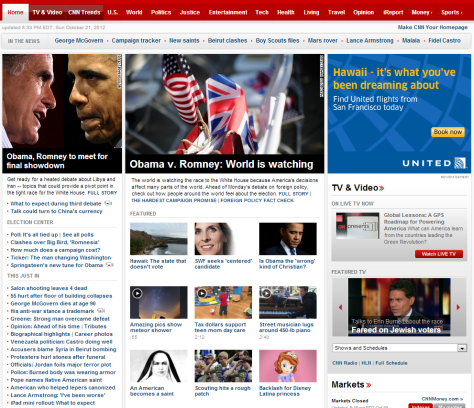This image is a detailed screenshot of a CNN news website taken on Sunday, October 21st, 2012, at 8:33 p.m. Eastern Daylight Time. The top of the image features a red navigation bar with the "Home" section highlighted in white text with a red background. Other sections such as "TV & Video" and "CNN Trends" are presented in a darker maroon color, while additional categories including "U.S.", "World", "Politics", "Justice", "Entertainment", "Tech", "Health", "Living", "Travel", "Opinion", "iReport", "Money", and "Sports" are displayed against a brighter red background.

Beneath the navigation bar, a banner titled "In the News" presents various trending topics listed as "George McGovern," "Campaign Tracker," "New Saints," "Beirut Clashes," "Boy Scout Files," "Mars Rover," "Lance Armstrong," "Malala," and "Fidel Castro."

Prominent headlines displayed on the page include "Obama, Romney to Meet for Final Showdown" and "Obama vs. Romney: The World is Watching," capturing the anticipation surrounding the upcoming presidential debate.